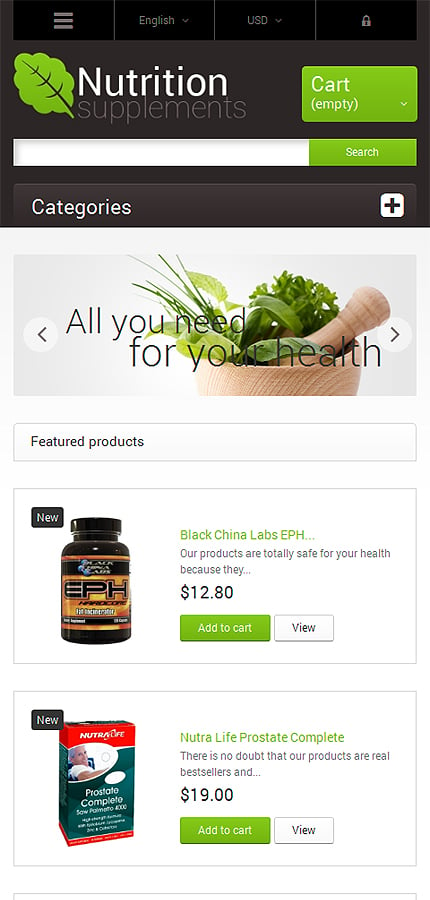The image appears to be a vertical, narrow screenshot from a mobile nutrition supplement website. At the very top, there is a gray header with the text "Nutrition" in white, followed by "Supplements" underneath it. A green leaf icon is positioned on the left side of the header, while a green rectangle on the right displays "Cart empty." Below this, there's a search bar which is white on the left side and green on the right, with the word "Search" displayed on the green portion.

Following the search bar, the word "Categories" is written in white text, next to a white square with a black plus symbol on the right. Below this section, there is a gray rectangle featuring an image of a wooden bowl with a wooden pestle, filled with various greens like lettuce and herbs. The text "All you need for your health" is displayed over this image, with navigation arrows on either side.

Underneath the promotional graphic, there is a section titled "Featured Products." The first featured product is displayed in a rectangle, showcasing a black bottle with a yellow-brownish label. The bottle is labeled "EPH" with a "new" tag, and described as "Black China Labs EPH. Our products are totally safe for your health because they..." priced at $12.80. Below this description, there is a green "Add to cart" button and a white "View" button.

The second featured product is housed in another rectangle. It features an image of a box labeled "Nutrilife Prostate Complete" with a picture of an elderly person on it. The description reads, "Nutrilife Prostate Complete. There is no doubt that our products are real bestsellers and..." priced at $19.00. This product also includes a green "Add to cart" button and a white "View" button on the right.